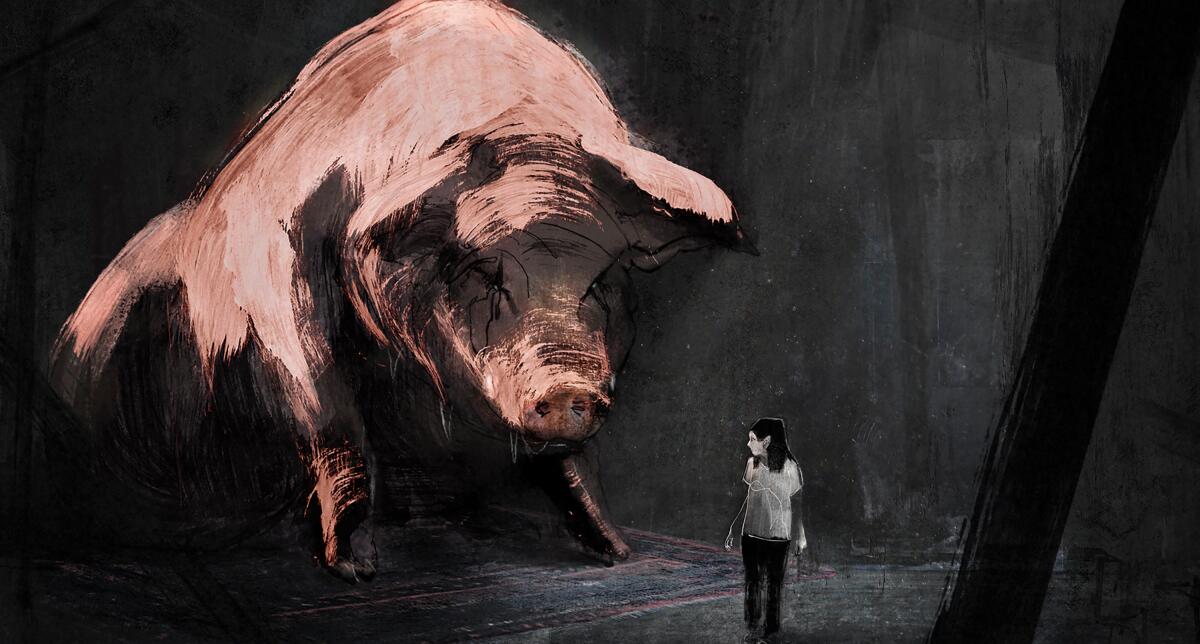This is a vividly detailed and dark-toned drawing that resembles a comic book illustration. Dominating the left side of the image is a colossal pink pig, significantly larger than the woman positioned slightly to the right of the center. The pig, with black streaks resembling tears running from its eyes, is propped up on its front legs while its hind legs and bottom rest on a carpeted floor adorned with black and red lines. The background is a deep charcoal gray mixed with black, adding to the moody atmosphere. The woman, who appears to be small in comparison, has dark hair and is dressed in dark pants and a light-colored t-shirt. She faces away from the pig, looking over her right shoulder directly at it. The pig gazes back at her with a blank expression, creating a haunting and surreal interaction. Both figures seem to be in a dark, ambiguous space, possibly a desolate building suggested by a black streak to the far right that could imply a fallen beam or mere texture in the artwork.